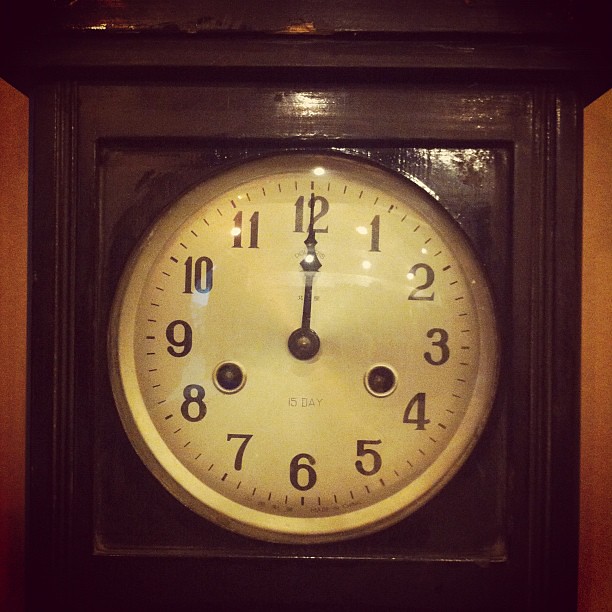The image depicts an old, weathered grandfather clock with a dark brown wooden body and base. It has a creamy off-white clock face adorned with black numerals and dash markings around the circumference. The clock indicates the time is precisely 12 o'clock, with both the hour and minute hands pointed at the 12, partially obscuring the maker's mark. Prominently displayed on the clock face is the notation "15 day." Notably, there are two small, dark brown circles positioned near the 4 and 8 numerals, whose purpose is unclear. The clock's wooden frame reflects a bit of light, enhancing the visible grain of the dark wood. The background features an orangey-brown, burnt umber wall, adding warmth to the overall scene.